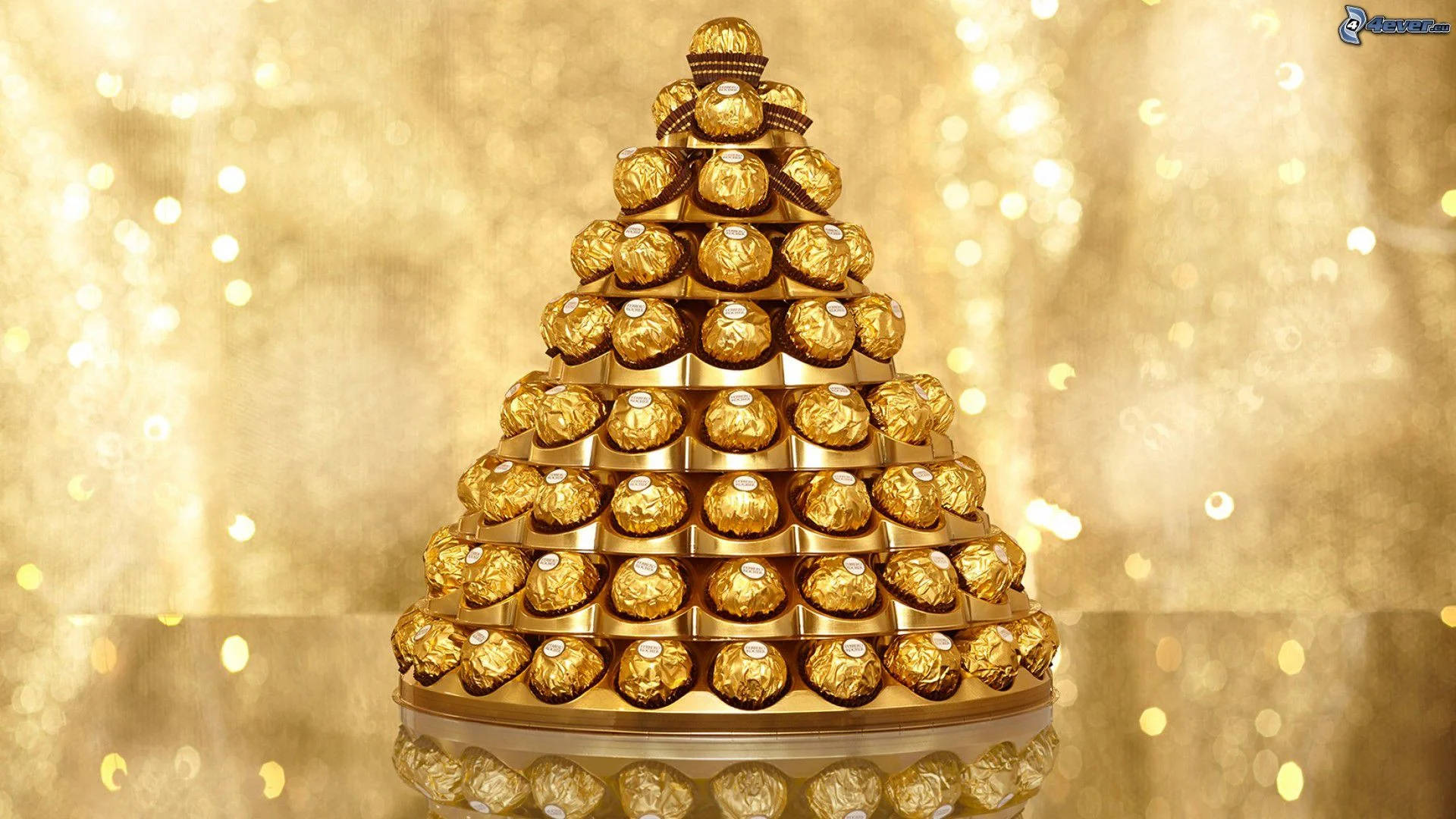The promotional photograph showcases an elegant display of round chocolate bars and gold-foil wrapped chocolate balls, likely Ferrero Rocher, arranged in a conical, tower-like stand. The tower mimics the shape of a Christmas tree, with wider rows at the base that gradually taper off towards the top, each row containing fewer chocolates until the apex where a single chocolate ball is perched. The chocolates, presented in dark brown bases with white dots and small white stickers on top, sit neatly in indentations on each row of the shimmering gold cone. This luxurious arrangement is placed on a highly reflective, flat metal surface, amplifying its dazzling appearance. The backdrop features a rich, gold fabric adorned with bright, sparkling dots, harmonizing with the overall opulent theme of the display, intended to captivate potential buyers.